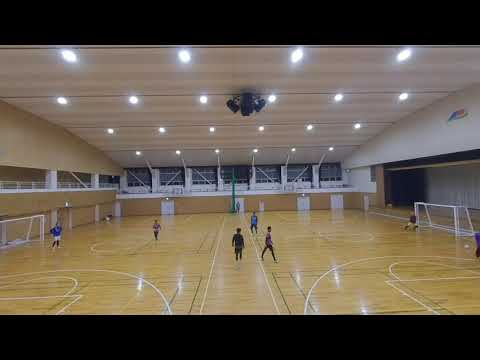Inside a multipurpose gymnasium with a light blonde wood floor prominently marked with white basketball lines and green badminton lines, several people are scattered across the court. White soccer goals stand on both the left and right sides, easily identified by their white netting. Among the individuals, one person in dark clothing can be seen walking towards the back of the court, while another in a purple shirt with black pants is heading to the right. The ceiling, lined with staggered grey and white beams, features six rows of white lights and a central black apparatus. The left wall is divided into a brown lower section, a mid-level white barrier leading to an upper level with light brown seating, and a large opening. The far back wall transitions from brown at the bottom to a white strip midway, culminating in a row of windows, with only the center window slightly open. On the right side, a stage-like overhang is present, with a heavily shadowed black square opening below it. The entire image is framed by thick black borders at the top and bottom, accentuating the detailed, dynamic scene within the gym.